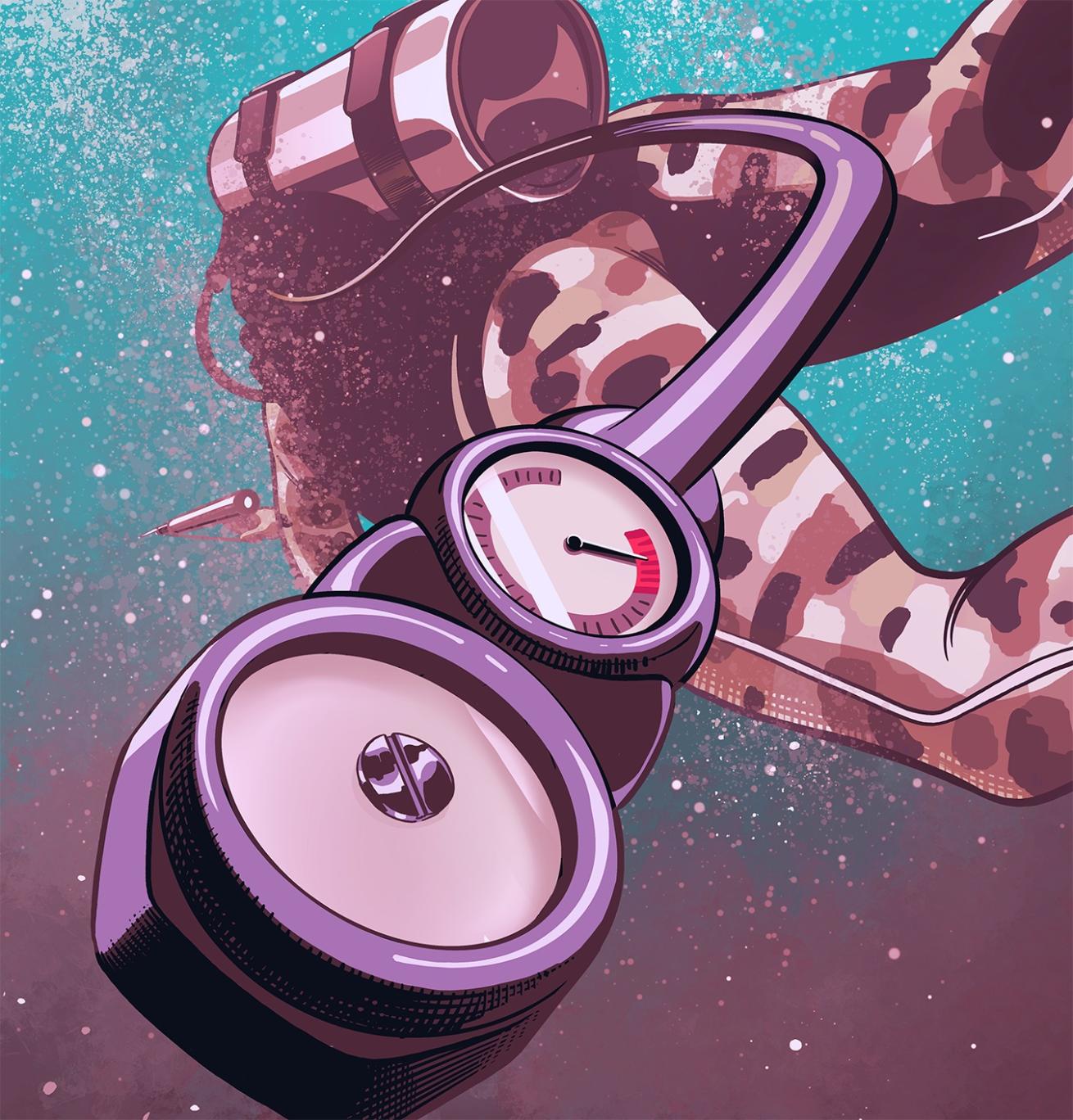This artwork portrays an underwater scene featuring a scuba diver armed with a harpoon gun. The diver, seen from behind, is dressed in a camouflage wetsuit with a mix of brown, black, beige, white, gray, and slight hints of green, resembling jungle or desert patterns. The water surrounding the diver transitions from a light sea green-blue gradient at the top to a chalky red at the bottom quarter, creating a visually striking background. Scattered throughout the water are debris and numerous white and silver spots representing air bubbles. The diver's equipment includes a silver air tank on their back, from which an air line extends to a floating mouthpiece. The attached gauge, with a black needle pointing to the red area, indicates low oxygen levels, suggesting the diver needs to surface soon. The diver's right hand is extended, aiming a harpoon gun towards an unseen target, adding an element of tension and mystery to the scene.